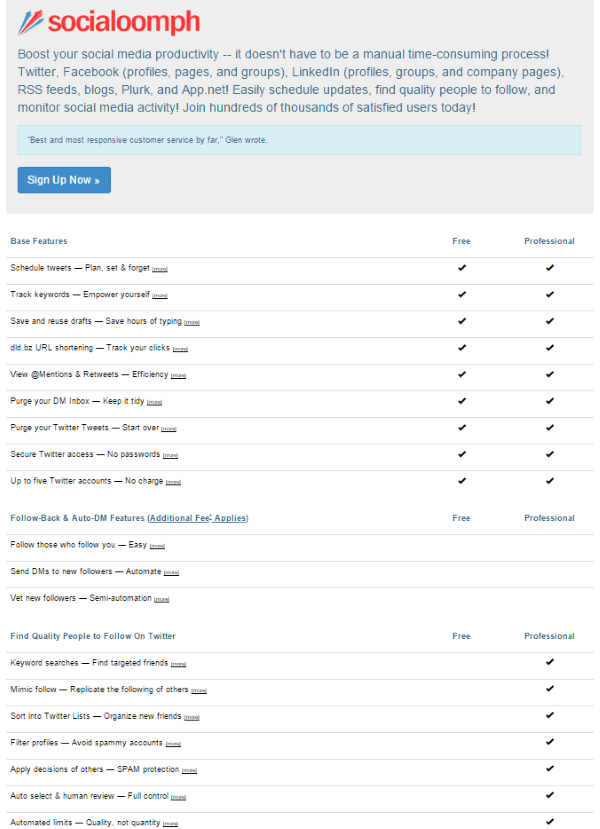At the top of the image, there is a light bluish-gray bar extending about a quarter of the way down. In the upper left section of this bar, there are three arrows (two blue and one red) arranged like fireworks pointing towards the upper left corner. The text within this section includes the brand name "Social Oomph" in red, followed by gray text that reads: "Who's your social media productivity? It doesn't have to be a manual time-consuming process. Twitter, Facebook Profiles, Pages and Groups, LinkedIn Profiles, Pages, Groups, and Company Pages, RSS Feeds, Blogs, Plurk, and App.net. Easy Scheduling Updates, Find Quality People to Follow, and Monitor Social Media Activity. Join Hundreds of Thousands of Satisfied Users Today."

Below this, within a bluish box, there is black text stating: "The Best and Most Responsive Customer Service By Far, Glenro." At the bottom left of the image, there is a prominent blue button with white text that reads: "Sign Up Now."

The lower section of the image features a list of "Base Features," which are divided into free and professional categories. All text in this section is black, and the right side of the list is marked with black check marks. The base features include: "Schedule Tweets," "Track Keywords," "Save Stuff," etc., available in both the free and professional plans. However, "Auto Follow" is listed but not included in either plan, raising the question of why it is even advertised.

Under "Quality People," the features listed are available only in the professional plan and include: "Keyword Searches," "Mimic Files," "Sort into Twitter Lists," "Filter Profiles," and additional unspecified features indicated by "Profile something, something, something."